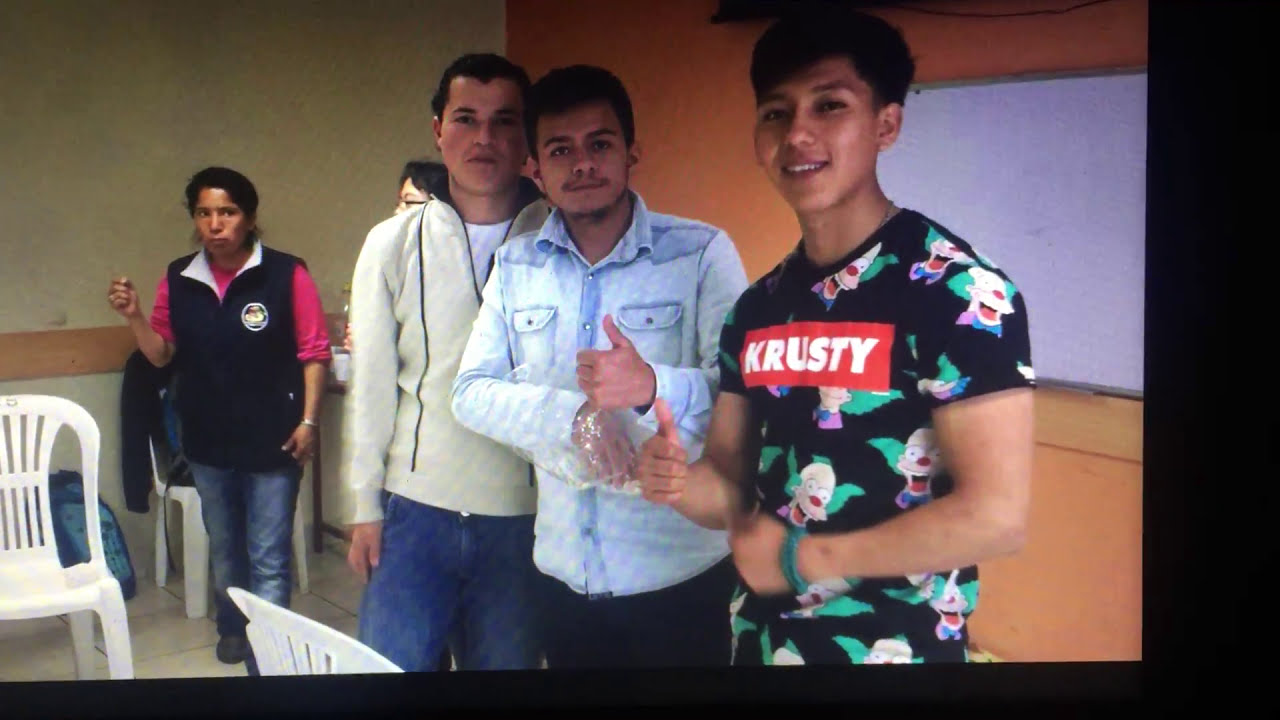The image depicts an indoor setting that appears to be a classroom or presentation room, characterized by tile flooring and a mix of wall colors, including an orange wall with a whiteboard and a light-colored wall with wood trim. In the bottom left corner of the image, there are a couple of plastic lawn chairs. Central to the image is a group of five people, most of whom are looking at the camera. Notably, the three individuals in the front center are the main focus: one man, wearing a black shirt adorned with heads of Krusty the Clown from The Simpsons and a red emblem reading 'Krusty', gives a thumbs-up with his right hand; another individual, wearing a light blue jacket or long sleeve shirt and dark pants, also gives a thumbs-up while holding what appears to be a plastic bag in their other hand; the third person, in a white hoodie and blue jeans, stands to their left with his arms at his sides. Additional figures include a person in a black vest, pink shirt, and blue jeans, whose right arm is raised slightly, and a partially visible person with glasses and black hair in the background. The people are positioned centrally, while the dry erase board is situated in the upper right of the image. The scene is accentuated by various colors: tan, brown, white, green, red, blue, light blue, pink, and purple.